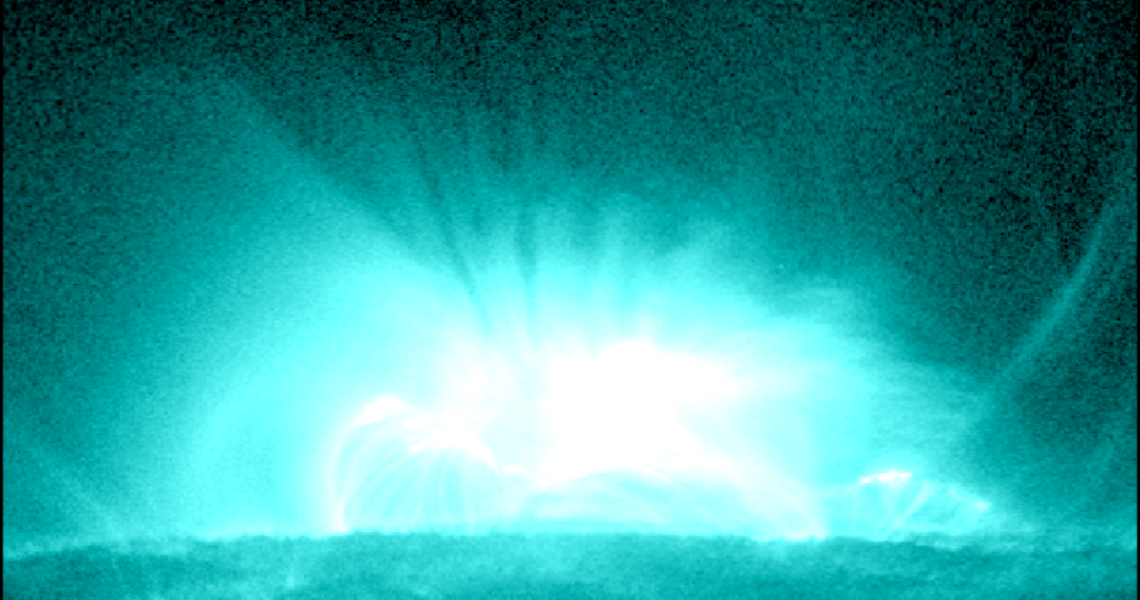The image depicts a low-resolution, abstract scene dominated by a bright, bluish-green light source, potentially resembling an explosion. The central focus is a vivid, intense blue-teal burst of light, surrounded by fuzzy black dots at the top. The surrounding colors transition from white at the core to greenish hues, and finally to a more prominent blue towards the edges. The bright light appears to shift the atmosphere and magnetic field, creating a surreal effect. The background is mostly black, and the bottom portion of the image is ambiguous, possibly representing a land or water area. The image's overall fuzziness and lack of clear detail make it difficult to determine its exact nature, giving the impression of an overexposed photograph or a still from a movie scene.